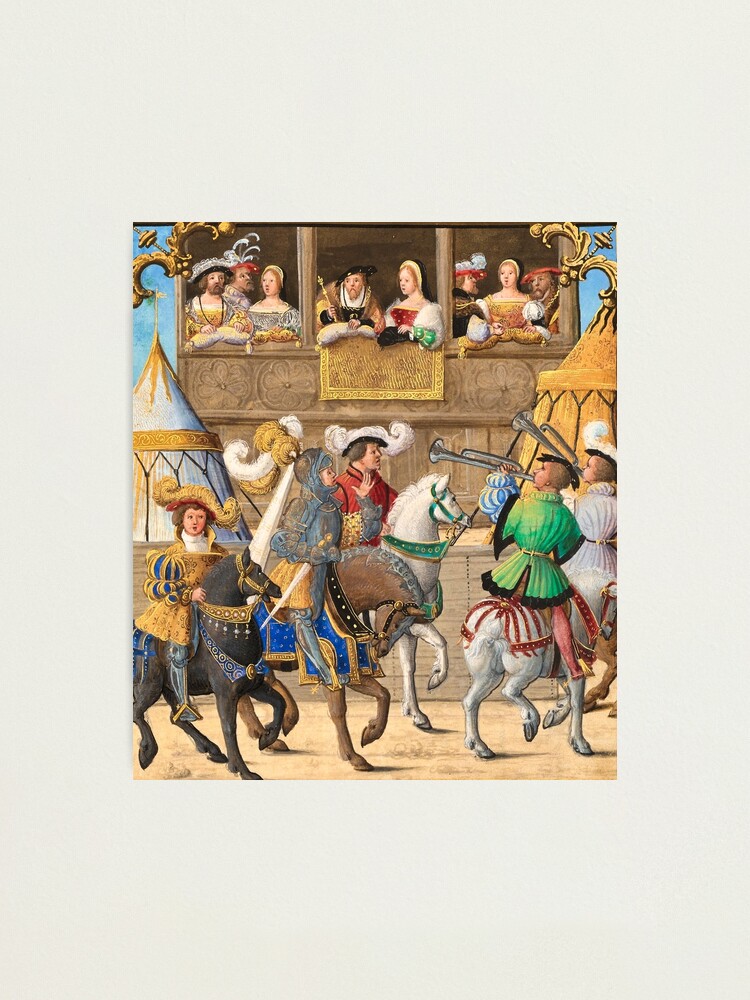The image showcases a Renaissance-era painting set against a gray background, featuring a central scene bustling with activity and rich detail. In the foreground, multiple figures ride horses in an arena of dirt. Among them, a nobleman in a golden outfit and hat commands attention on a black horse, while a knight clad in armor with a golden white-plumed helmet rides a brown horse adorned with blue trappings. Nearby, a man in a red jacket and white hat guides a white horse, and a figure in a green jacket with a red-belted white horse plays a trumpet, adding to the scene's vibrant dynamism.

The background reveals a built-up stage or viewing platform where wealthier spectators, possibly including a regal king and queen in lavish black and white attire, observe the event below from luxurious, tented seats decked in gold and white. The overall scene conveys an atmosphere of grandeur and opulence, capturing a lively, celebratory moment from a bygone era.